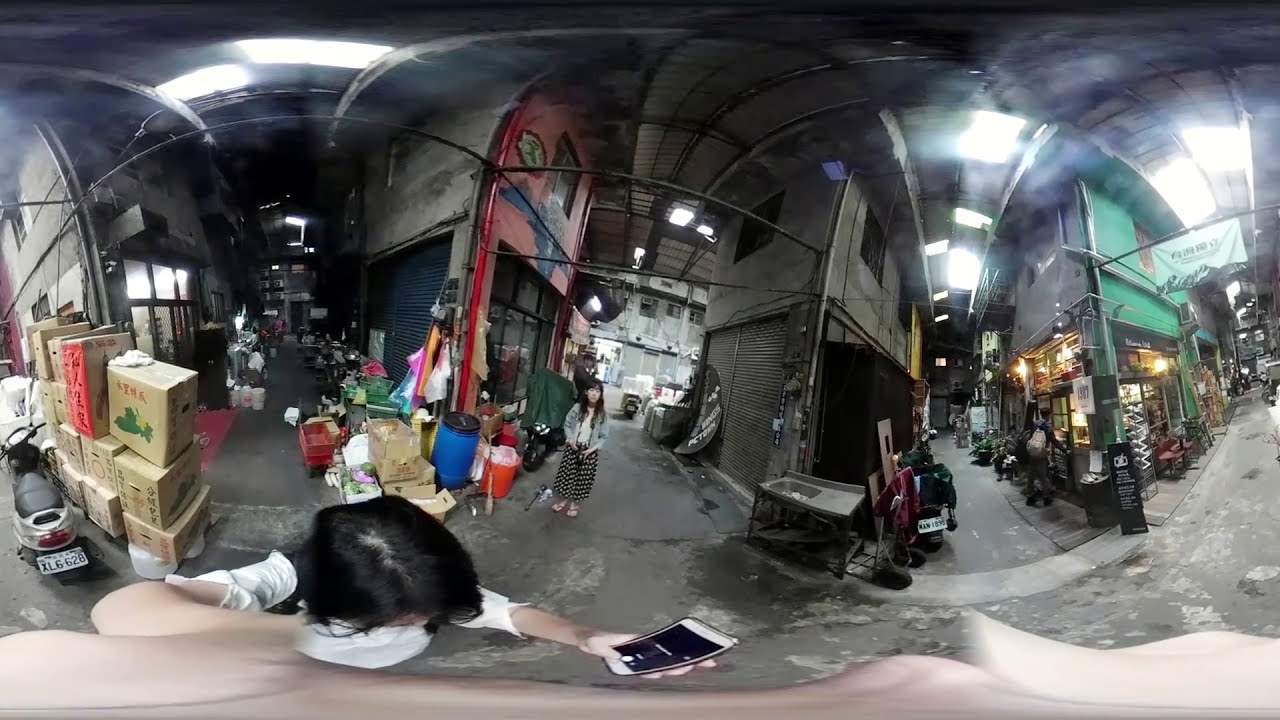The image depicts a cluttered, industrial shopping area or warehouse-like setting captured in a 360-degree panoramic shot. In the forefront, a woman with black hair and light skin stands close to the camera, holding up her smartphone. She wears a white long-sleeve shirt and stands off to the left side of the image. Behind her, another woman, seemingly of Asian descent, with long dark hair, is wearing a jean jacket, a black polka dot skirt, and sandals. This second woman is looking towards the camera.

The scene features numerous storefronts and walkways lined with merchandise and clutter. To the left, there is a motorbike with a license plate and several cardboard boxes piled up. Directly behind the women, various metal buildings and roll-up metal doors, indicative of small shops, are visible. To the right, a pathway leads to a corner shop with a black facade on one side and a green exterior with a black sign on the other side, both illuminated with exterior lights. A flag sign protrudes from the building, emphasizing its status as a shop. The ground is concrete, adding to the industrial feel of the area, which is cluttered with goods and products for sale, suggesting a busy, albeit messy, shopping environment.